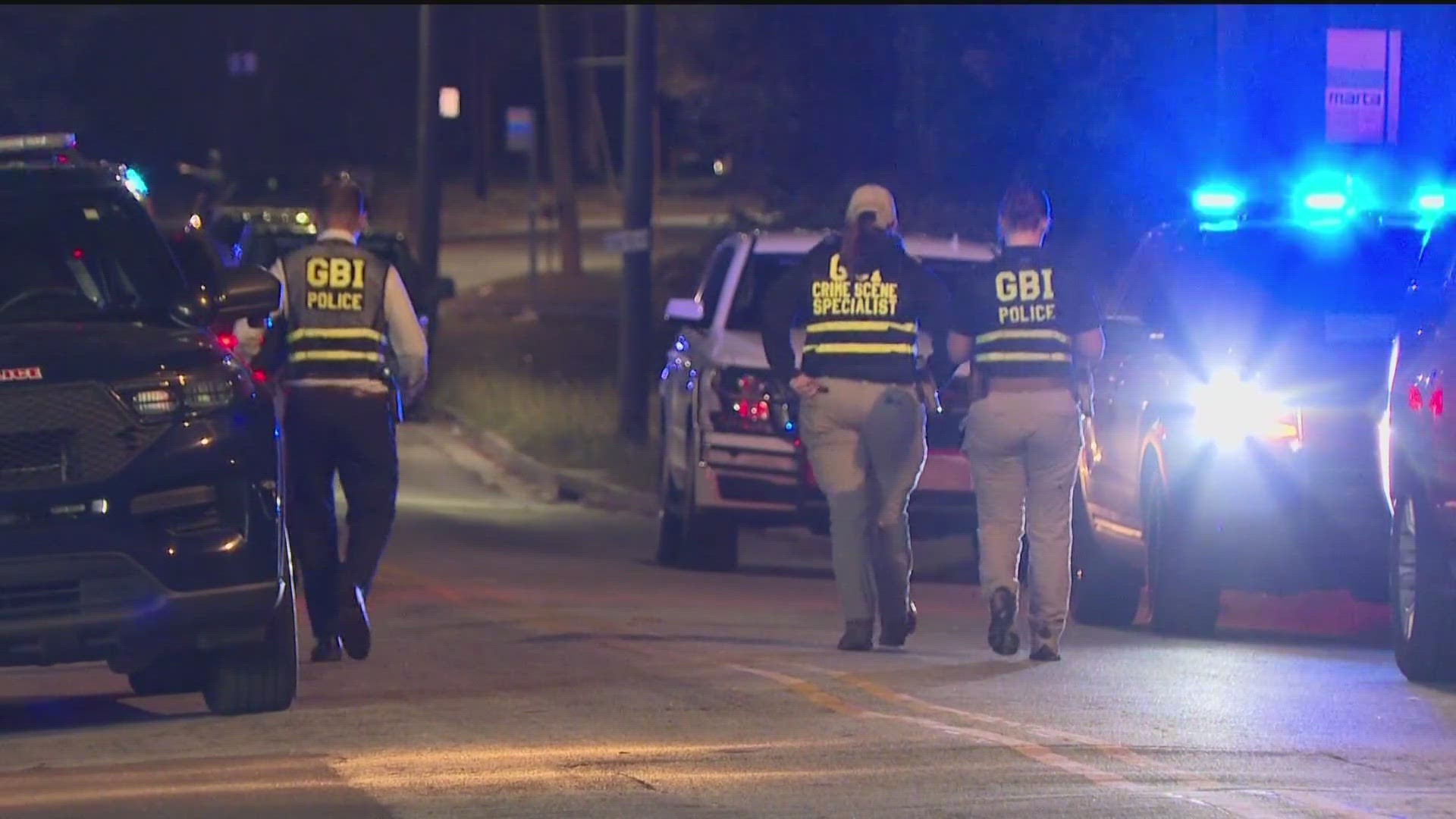This image depicts a nighttime urban scene with three law enforcement officers walking away from the camera, their backs facing us. Each officer is wearing dark-colored attire with high-visibility yellow lettering. The officer on the left is labeled "GBI Police," the middle officer is identified as "GBI Crime Scene Specialist," and the right officer also bears the label "GBI Police." Their vests feature two horizontal yellow stripes below their designations. To the sides of the street, numerous vehicles are visible, including several police cars with blue and white lights flashing on the right side and other civilian cars. Yellow lines mark the gray pavement, and a patch of green-brown area is visible ahead. On the right in the background, a sign reads "MARTA," while the left side reveals some lit buildings amidst the darkness. The top of the image is predominantly black, indicating the night sky or a shadowed area.